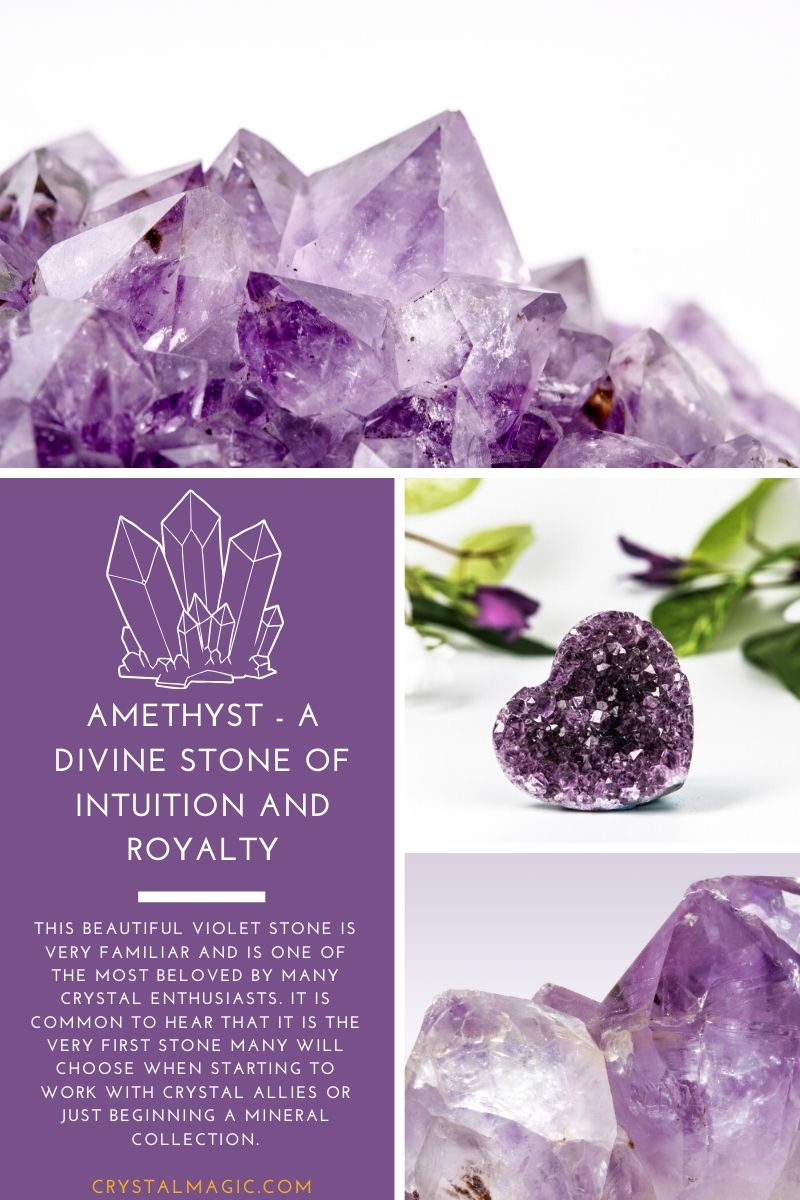This digital advertisement prominently features an enticing showcase of amethyst, emphasizing its esteemed place among crystal enthusiasts. The top third of the flyer is dominated by a large, captivating close-up photograph of purple amethyst gems, highlighting their intricate crystalline structure and rich violet hues. Divided vertically, the bottom two-thirds hold two smaller photographs on the right side: one displaying a heart-shaped amethyst stone sitting on a white surface, and another providing an even more detailed close-up of amethyst's majestic texture. The left side of this section is a solid purple block adorned with an illustration of gemstones. This area contains the textual description: "Amethyst, a divine stone of intuition and royalty." Further, it elaborates, "This beautiful violet stone is very familiar and is one of the most beloved by many crystal enthusiasts. It is common to hear that it is the first stone many will choose when starting to work with crystal allies or just beginning a mineral collection." The advertisement concludes with crystalmagic.com, inviting viewers to explore more about this enchanting stone.